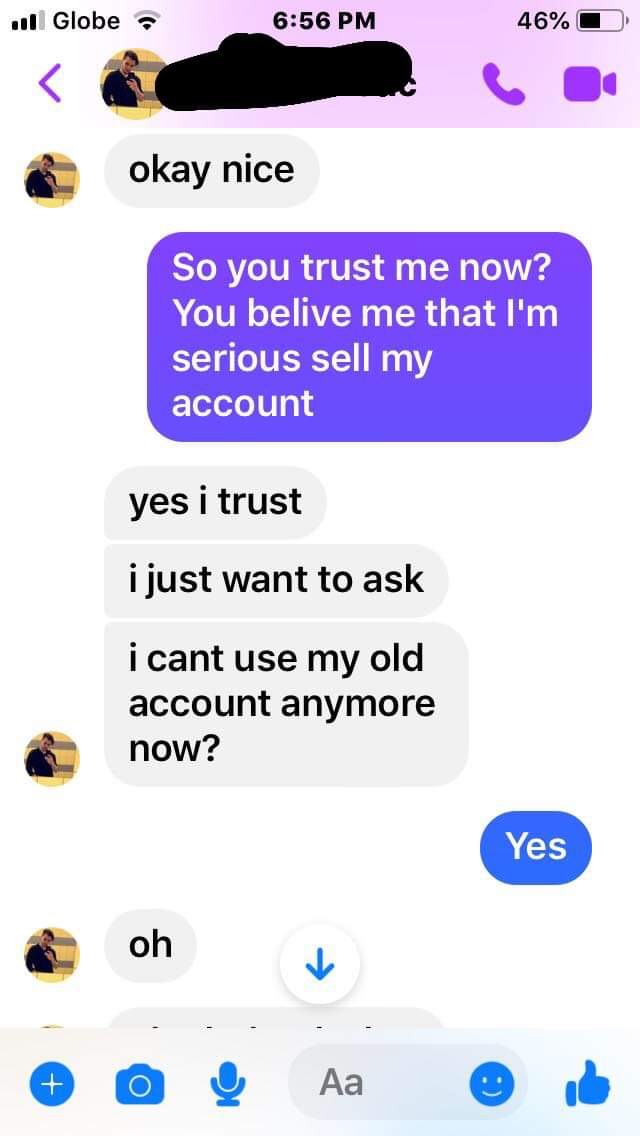This is a detailed screenshot from an iPhone displaying a Facebook Messenger conversation with a purple theme. The device's status bar shows the carrier as Globe, the time as 6:56 PM, and the battery at 46%. At the top, a pale purple rectangle with an icon of a man taking a picture in a mirror against a yellow and purple wall is visible, with his name obscured by black marker for privacy.

The conversation begins with a gray speech bubble on the left that reads, "okay nice." Below that, a large purple bubble on the right in white font reads, "so you trust me now? You believe me that I'm serious? Sell my account?" The thread continues with the left side responding in three gray speech bubbles: "yes, I trust," "I just want to ask," and "I can't use my old account anymore now?" Finally, a blue bubble on the right responds with "yes," followed by a gray bubble on the left reading "oh."

The bottom of the screenshot shows elements of the Messenger interface, including options for speech and emojis. Some additional responses appear cut off at the bottom of the image, indicating that more of the conversation exists further down.